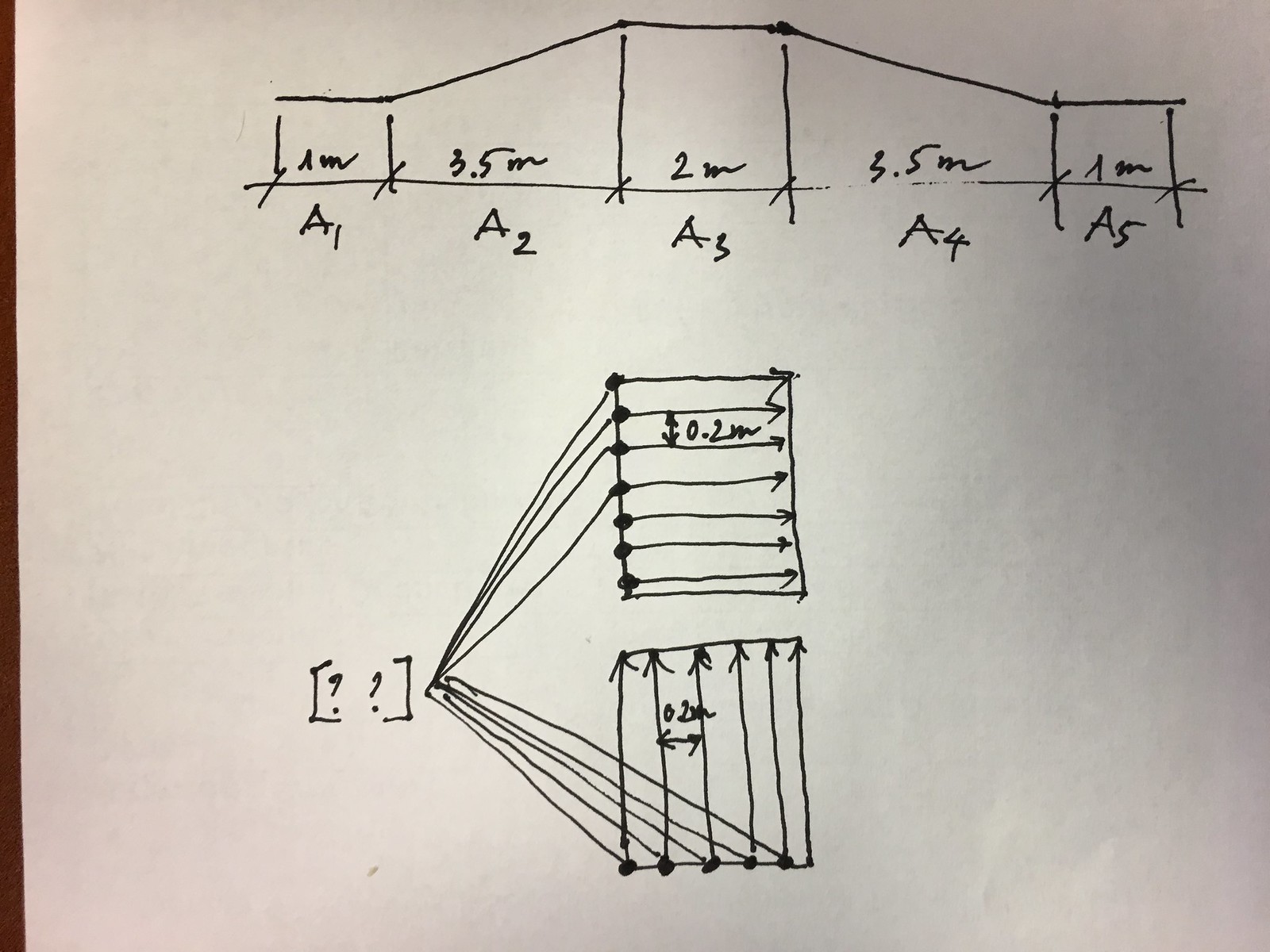This image features a detailed engineering line drawing. At the top of the image, a straight horizontal line is connected to another line that ascends at a 70-degree angle. This is followed by another straight horizontal line, forming a mound-like shape when the entire structure is mirrored. At the base of this configuration, several extension lines mark various points, labeled as A1, A2, A3, A4, and A5, indicating precise dimensions and measurements.

Below these labeled points, a series of converging lines create a perspective effect. These lines include five ascending and five descending, forming a focal point illustration. Adjacent to this section, there are dimension annotations encased in parentheses that read "??", indicating unspecified or unknown measurements. The overall diagram appears to be a technical sketch, possibly for an engineering or architectural project, showcasing detailed dimensional data and perspective alignment.